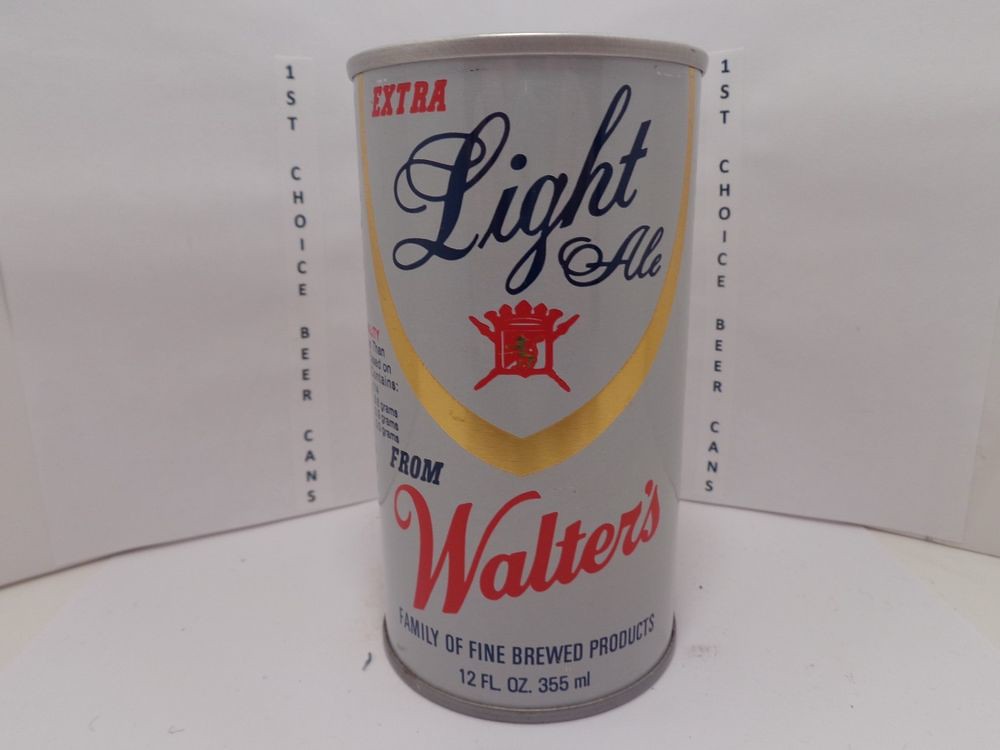The image displays a predominantly white surface featuring black text on both the left and right sides stating, "First Choice Beer Cans." Situated centrally between the text is a cylindrical beer can, providing a frontal view that obscures both the top and bottom of the can. The can itself showcases a detailed design: the top and bottom edges appear metallic, while the central area is wrapped in white packaging. 

In the upper left-hand corner of the can, the word "Extra" is prominently written in red. Directly below, "Light Ale" is written in blue. Adding a touch of visual complexity, a red emblem featuring swords extends from behind these words. Below the emblem, the phrase "From Waters" appears, with "From" in blue and "Waters" in red. At the bottom portion of the can, the text "Family of Fine Brewed Products" is displayed in blue, followed by "12 FL. OZ." and "355 ML" in smaller blue font beneath it.